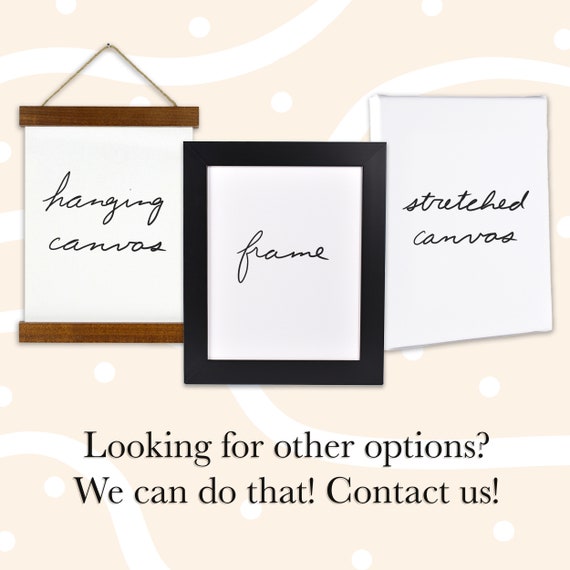The image showcases an advertisement featuring three canvases presented in distinct styles, arranged in a row from left to right against a yellowish background with white curvy lines and circles. The first canvas on the left, labeled "hanging canvas," is suspended by a brown rope, anchored by a nail on the wall. It features a wooden frame on both the top and bottom edges and is written in italicized cursive. In the middle, the second canvas is encased in a simple black frame and labeled "frame." The third canvas on the right, labeled "stretched canvas," appears as a plain, white stretched canvas, also with cursive text. Below these canvases, there is a message in black serif font that reads, "Looking for other options? We can do that. Contact us!" The overall color scheme includes beige, white, black, brown, and off-white, contributing to a digitally created aesthetic aimed at advertising framing services.